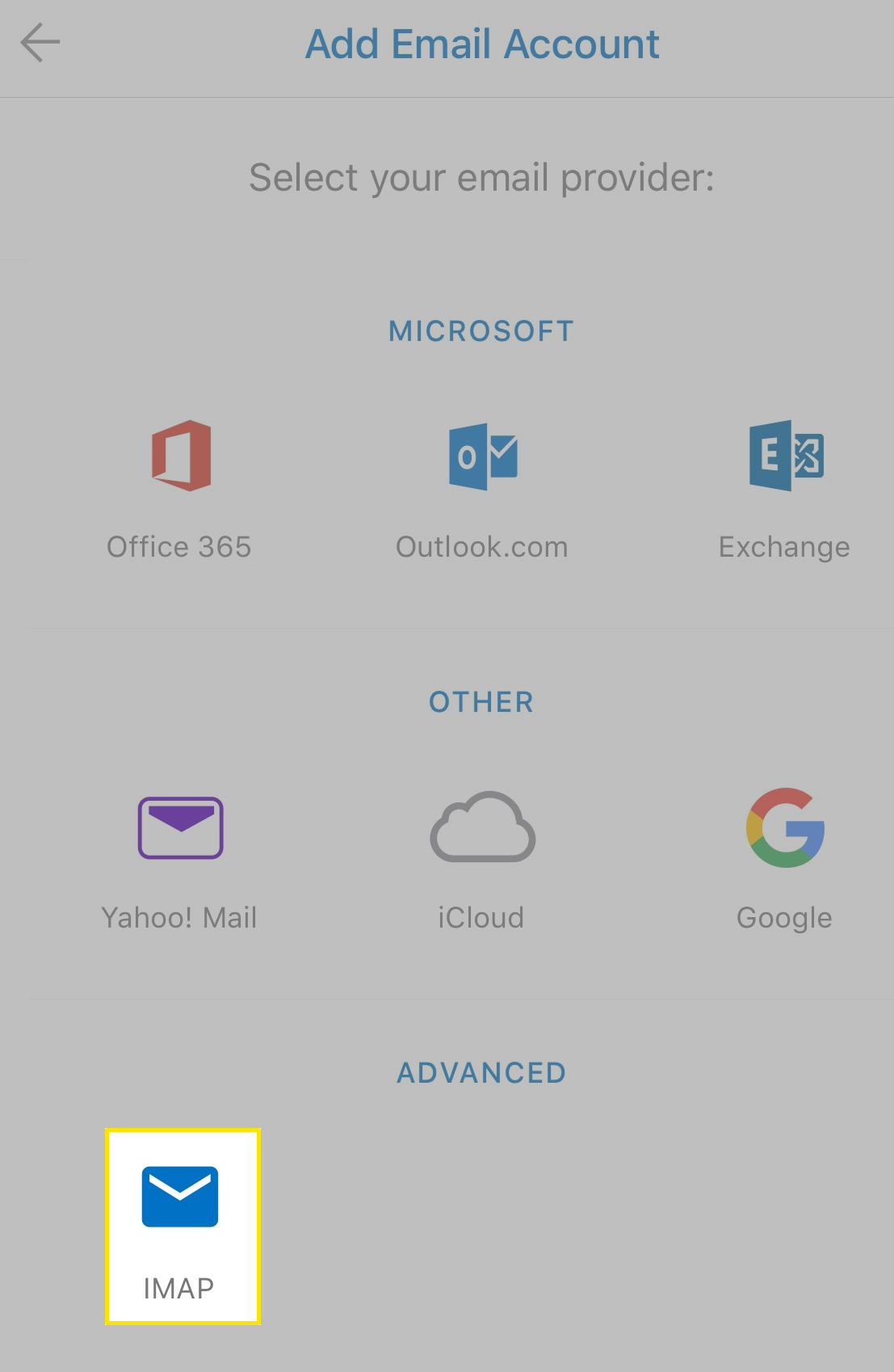This image is a screenshot showing the interface for adding an email account on a light gray background. At the top center, there is a black directional arrow pointing to the left. Directly below, in blue text, it says "Add Email Account." A faint gray line runs horizontally from left to right beneath this text.

Centered underneath the line, in black text, it reads "Select Your Email Provider." The interface then displays several selectable options:

1. **First Row:** 
   - A red-framed square with a white center, labeled "Office 365."
   - A square containing a circle in the middle with a blue envelope, labeled "Outlook.com."
   - A blue square with a white "E" icon, followed by a blue square with a crisscross emblem, labeled "Exchange."

2. **Second Row:**
   - A white envelope with a purple outline, labeled "Yahoo Mail."
   - A light gray outlined cloud labeled "iCloud.”
   - A multicolored "G" (red, yellow, green, and blue), labeled "Google."

Below these elements, centered blue text reads "Advanced."

In the bottom left corner, there is a white rectangular icon outlined in yellow featuring a blue envelope, with the text "IMAP" beneath it.